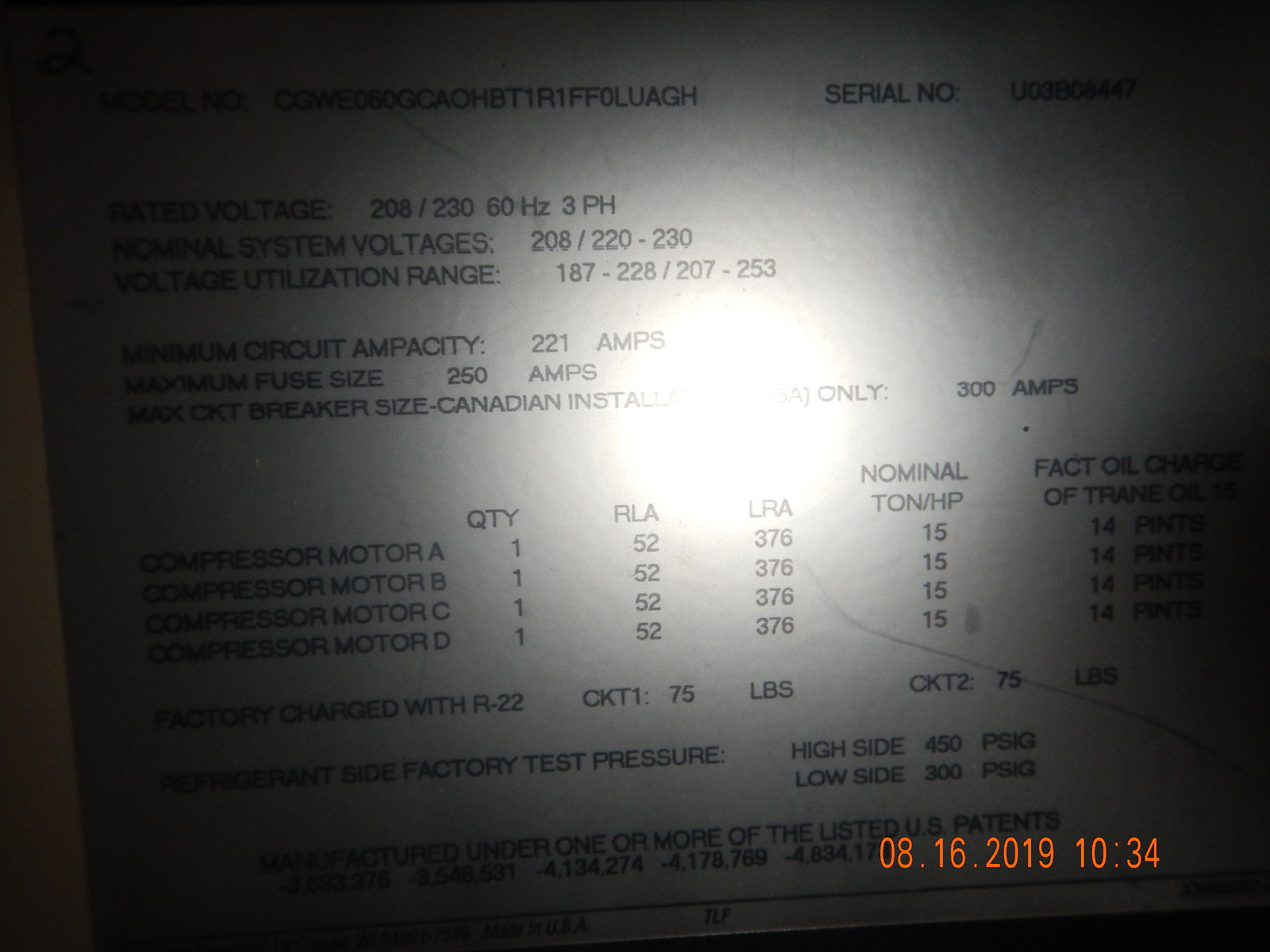The image depicts a detailed metal identification plate affixed to a piece of industrial equipment. At the very top of the plate, there are several illegible or garbled characters. Below this, a visible serial number reads "UD38." 

Further down, there are specifications related to the device's voltage ratings. It lists the voltage as 208/230 volts, with a frequency of 60 Hz, and a phase configuration of 3 pH. The plate specifies the normal system voltage as 208/220-230 volts.

Additionally, the voltage utilization ranges are provided: 187-228 volts and 207-253 volts, respectively. Lastly, the plate indicates the minimum circuit ampacity required for the device, which is 221 amps.